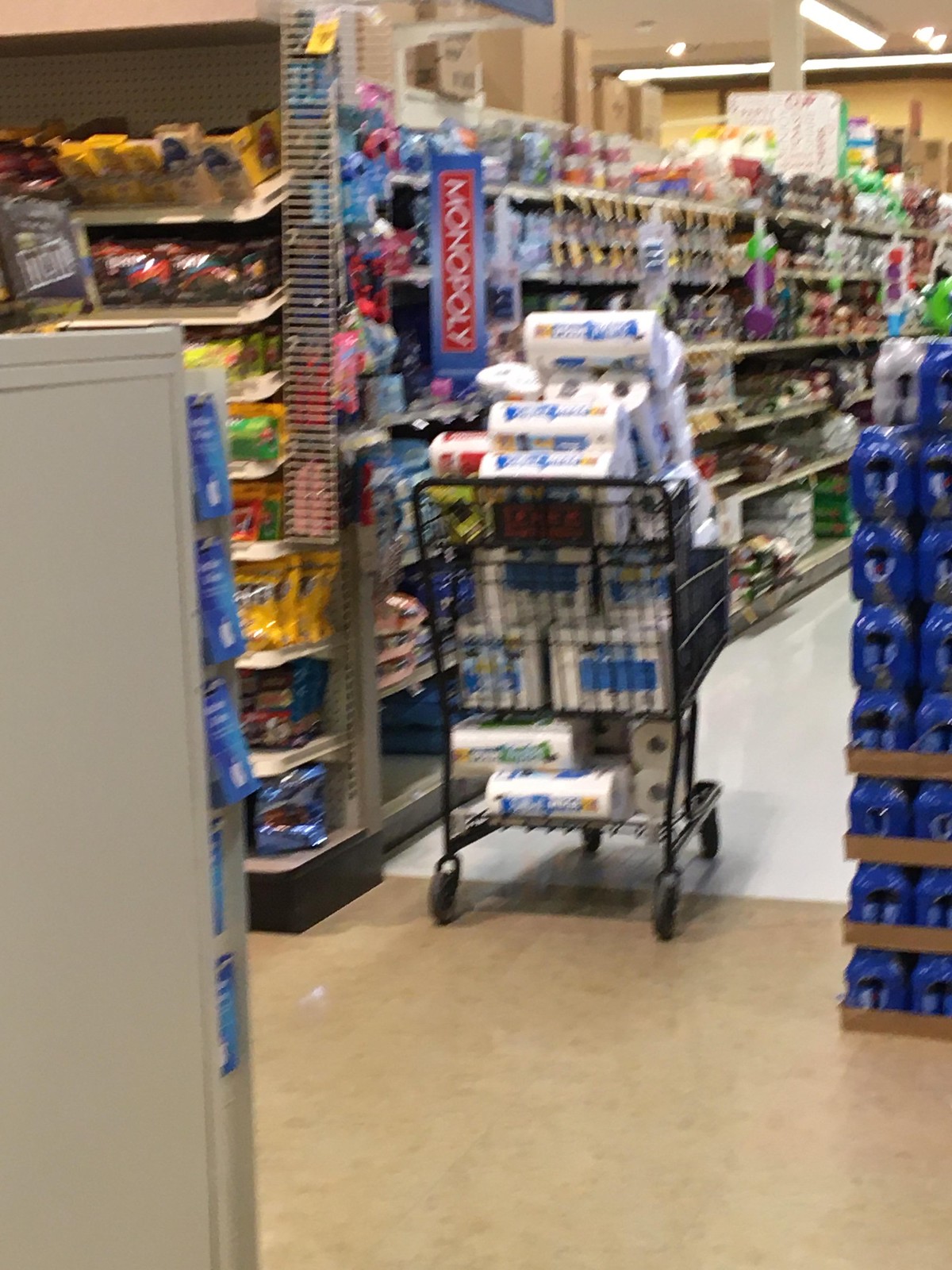Inside a bustling grocery store, a shopping cart is conspicuously overflowing with packages of toilet paper, reflecting a scene reminiscent of the 2020 lockdown rush. The cart, with its black frame and wheels, is packed high with rolls of toilet paper encased in white plastic wrapping, embellished with blue lettering. The backdrop is an aisle brimming with assorted items, including a stack of canned goods sealed in blue plastic on the right. On the left, a grey cabinet displays vertically hanging blue papers. A prominent vertical sign in the same aisle bears the word "Monopoly" in white text on a blue frame with a red border, hinting at a store promotion. Although no shoppers are visible, the image vividly captures a moment of pandemic-induced urgency through its central focus: a solitary cart overloaded with essential supplies.